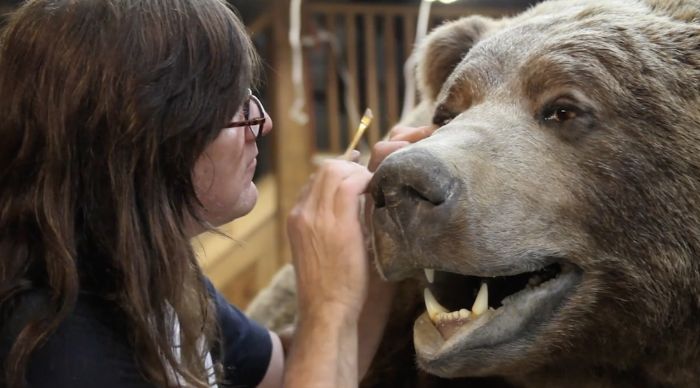This detailed color photograph captures a scene of a taxidermist, a Caucasian woman with long brown hair and glasses, meticulously working on a taxidermied brown grizzly bear. The woman is situated on the left side of the horizontally aligned image. She is wearing a short-sleeved navy blue shirt and is using a paintbrush to apply finishing touches to the bear, specifically focusing on the bear's right eye. Her other hand is gently adjusting the bear's eye area for precise detailing. The bear, occupying the right side of the photo, has a lifelike appearance with brown fur, brown eyes, a black nose, and a mouth displaying sharp teeth—two prominently large ones on the bottom and a single sharp tooth on the top. Notably, the bear's snout appears a lighter color compared to the rest of its face. The attentive expression of the woman contrasts with the bear's static, serene look. In the background, a wooden porch railing with vertical brown bars is visible, providing a rustic setting to this intriguing and detailed depiction of taxidermy work.